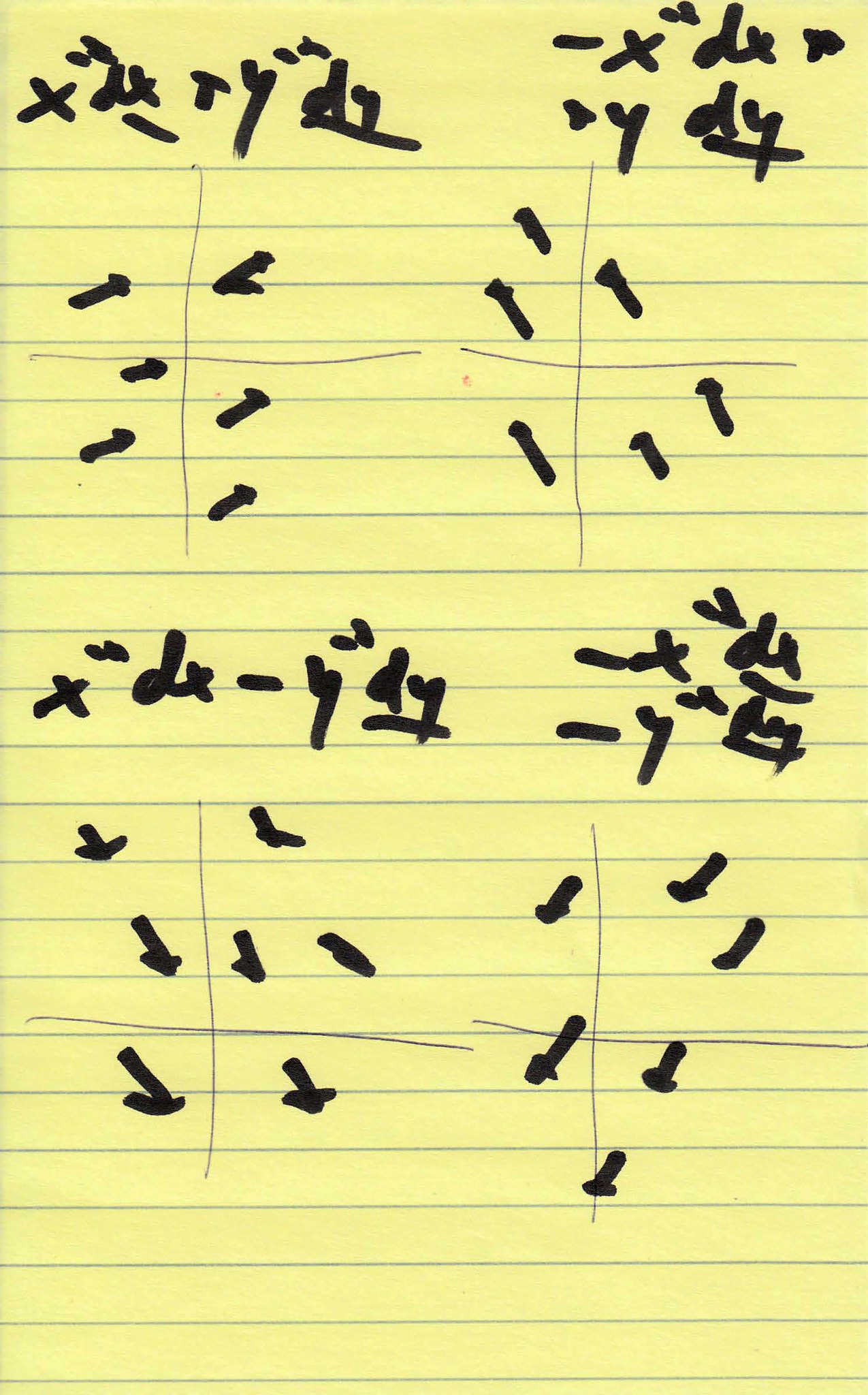This portrait-style image features a yellow background adorned with blue horizontal lines, mimicking lined paper. In the upper left corner of the paper, black marker notations read "X, DX, TY, DY," with "DY" underlined. On the top right, the text "-X DX +" can be seen. Beneath this, the words "= Y Y" are inscribed, with "DY" once again underlined. The image is divided into four main quadrants: top left, top right, bottom left, and bottom right. Each of these quadrants contains smaller cross patterns subdivided into four further sections. Within these sections, two or three straight marker lines are randomly oriented and distributed, giving the whole composition a chaotic yet structured appearance.